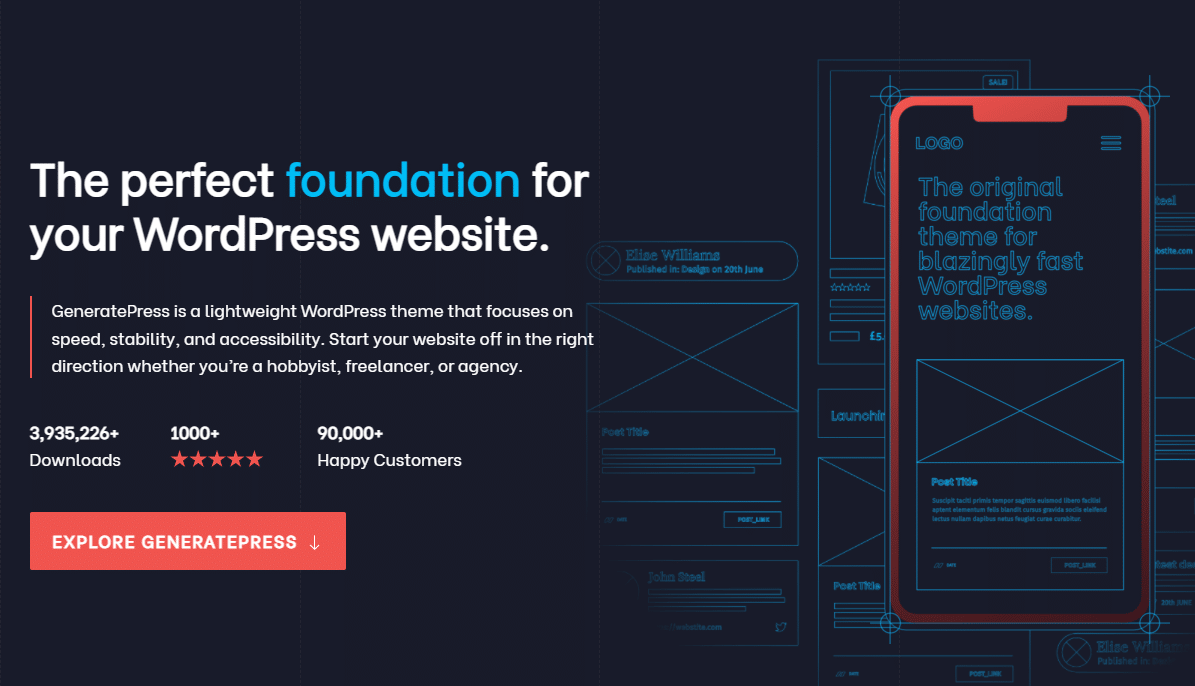The image is a horizontally-oriented screenshot with a solid black background. In the upper left corner, there is a prominent white text slogan in bold that reads, "The perfect foundation for your WordPress website," with the word "foundation" highlighted in blue. Just below this is a smaller, detailed description in white text: "GeneratePress is a lightweight WordPress theme that focuses on speed, stability, and accessibility. Start your website off in the right direction, whether you're a hobbyist, freelancer, or agency."

Further down, the image showcases impressive statistics: "3,935,226 downloads" is prominently displayed. To the right of this, it highlights "1,000+ Five Star Reviews" in red stars, and further to the right, it notes "90,000+ Happy Customers." At the bottom of the image is a vibrant red call-to-action button with white text that reads "Explore GeneratePress," accompanied by a white downward arrow.